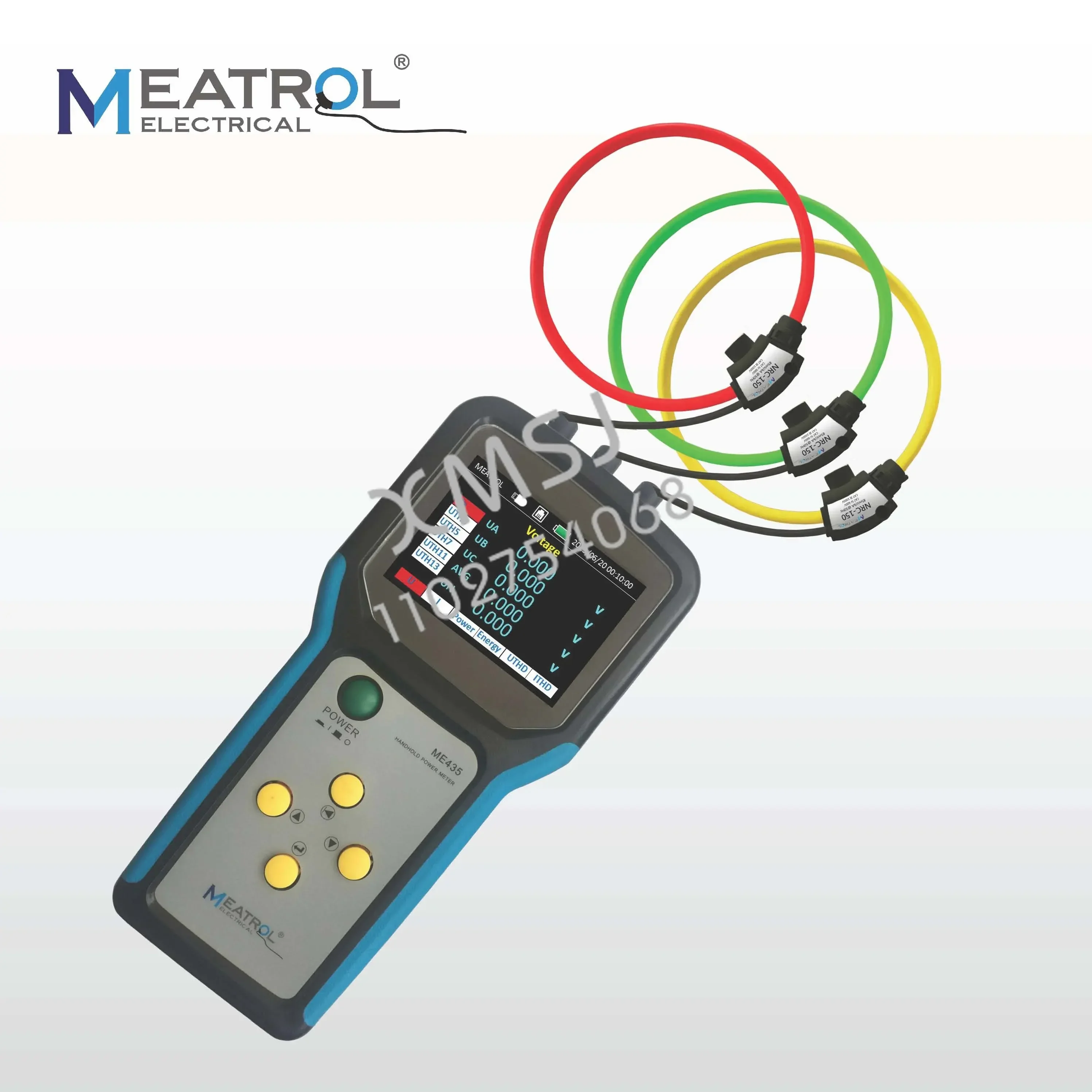This image is a detailed product photo of an electronic device branded "Mitra Electrical" in the upper left corner. The logo features a blue "M" and "O" with the "O" stylized to include a cord, spanning dark blue, light blue, and gray colors. Below the logo, "Electrical" is written in a small font. The device itself is predominantly black with blue borders and is situated centrally in the image. It has a digital color screen displaying various readouts including battery life, power, energy, UTHD, and ITHD, with the screen colors ranging from red, green, yellow, and blue to white. At the bottom of the device are four yellow buttons arranged to function as directional controls (up, down, left, right) and a green button labeled "Powered." Additionally, there are serial numbers on the device and three wires (red, green, yellow) emerging from its top. The device is also marked with the model number "ME435" and prominently features the name "Mitra."